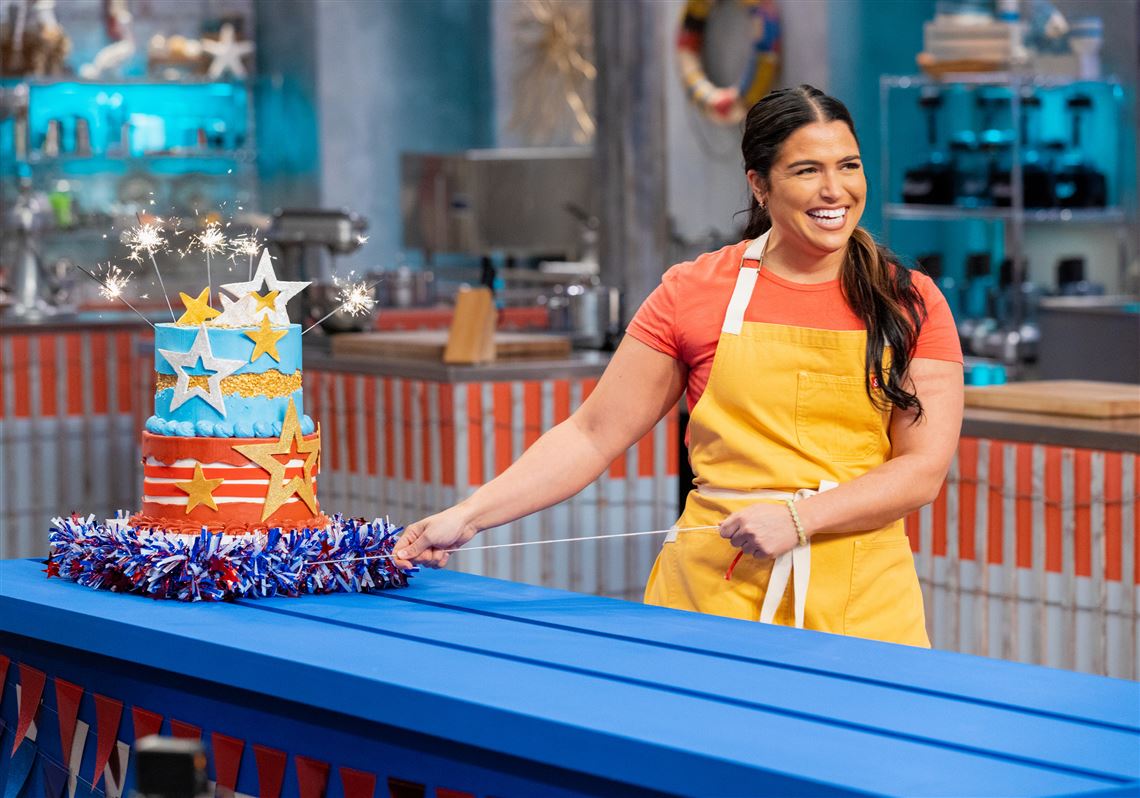In this vibrant, festive photograph, a woman stands proudly in a large, professional bakery, reminiscent of a cooking show setting. Her long black hair is elegantly pulled over her left shoulder, and she exudes joy with a wide, radiant smile. She is attired in an orange short-sleeve t-shirt paired with a yellow apron that ties at the waist and features white straps. A yellow bracelet adorns her left wrist. 

The woman is holding a string attached to a visually striking two-tier cake that celebrates the 4th of July. The cake sits on a blue counter and is adorned with intricate details: the bottom layer is orange with white stripes, while the top layer is blue, embellished with gold and white stars fastened elegantly around it. On top of the cake are sparklers that are lit and sparkling, accompanied by yellow and white stars. The cake is further decorated with fringe around its base, adding to its festive charm.

In the background, though slightly blurred, one can discern the bustle of a spacious kitchen. White and orange walls frame the scene, with coffee machines, cutting boards, various bakery items, and racks stocked with utensils and equipment contributing to the culinary environment. The overall ambiance of the image is one of celebration, meticulous craftsmanship, and the joy of baking.